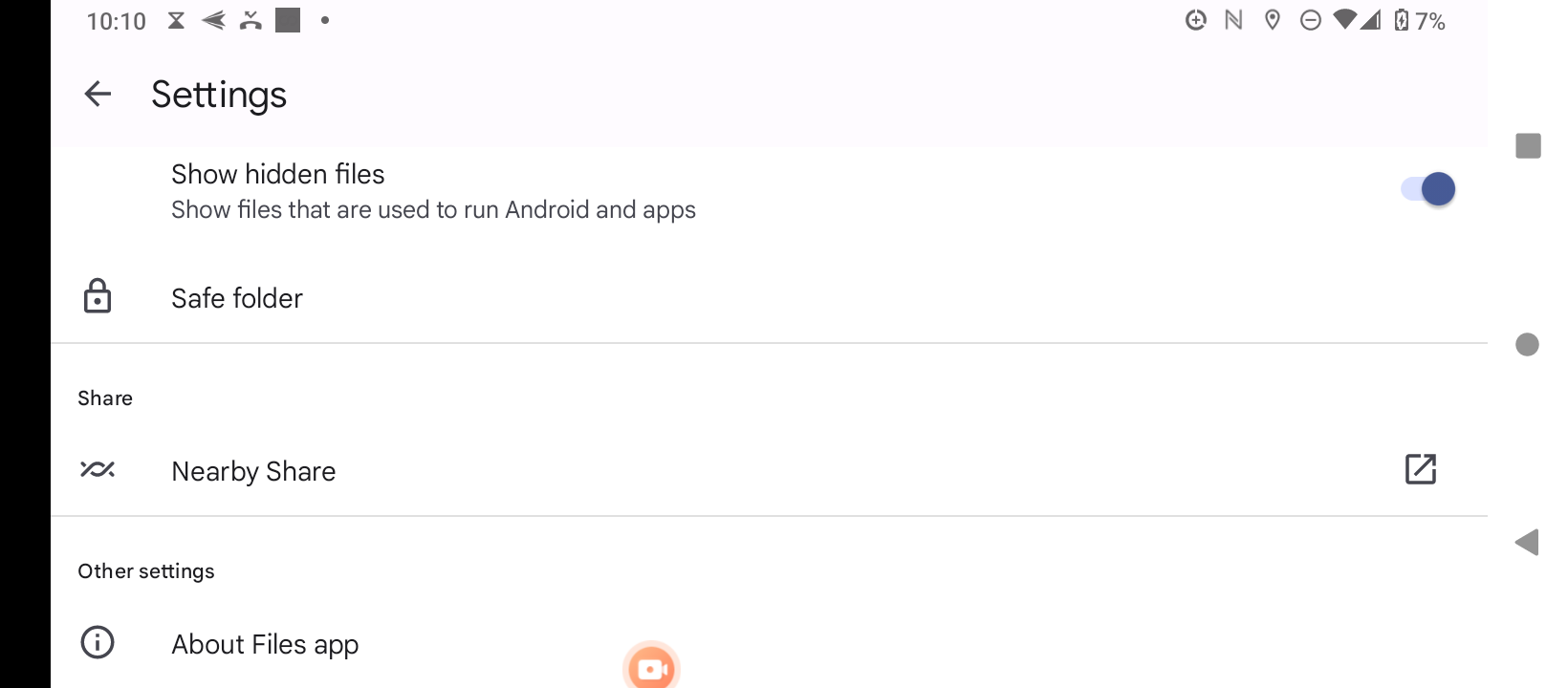A detailed description of the provided image would be as follows:

The image showcases an Android tablet's screen in landscape mode. At the top left corner, the time is displayed as 10:10. The top bar is populated with several icons: a hourglass shaped like two triangles, an arrow pointing to the left, a bone, and a black square. In addition, there are symbols indicating various functions, including a plus symbol, an "in" symbol, and a pointer symbol paired with a minus sign. On the right side of this top bar, connectivity icons are present along with the battery icon, which shows a 7% charge remaining. The screen also displays settings and airplane mode icons.

On the left side of the screen, there is a highlighted option labeled "Chosen files," indicating it is checked. At the bottom of the screen is a "Safe folder" along with options for "Share," "Nearby Share," and additional settings related to the file app. An orange camera logo is also visible near the bottom of the display.